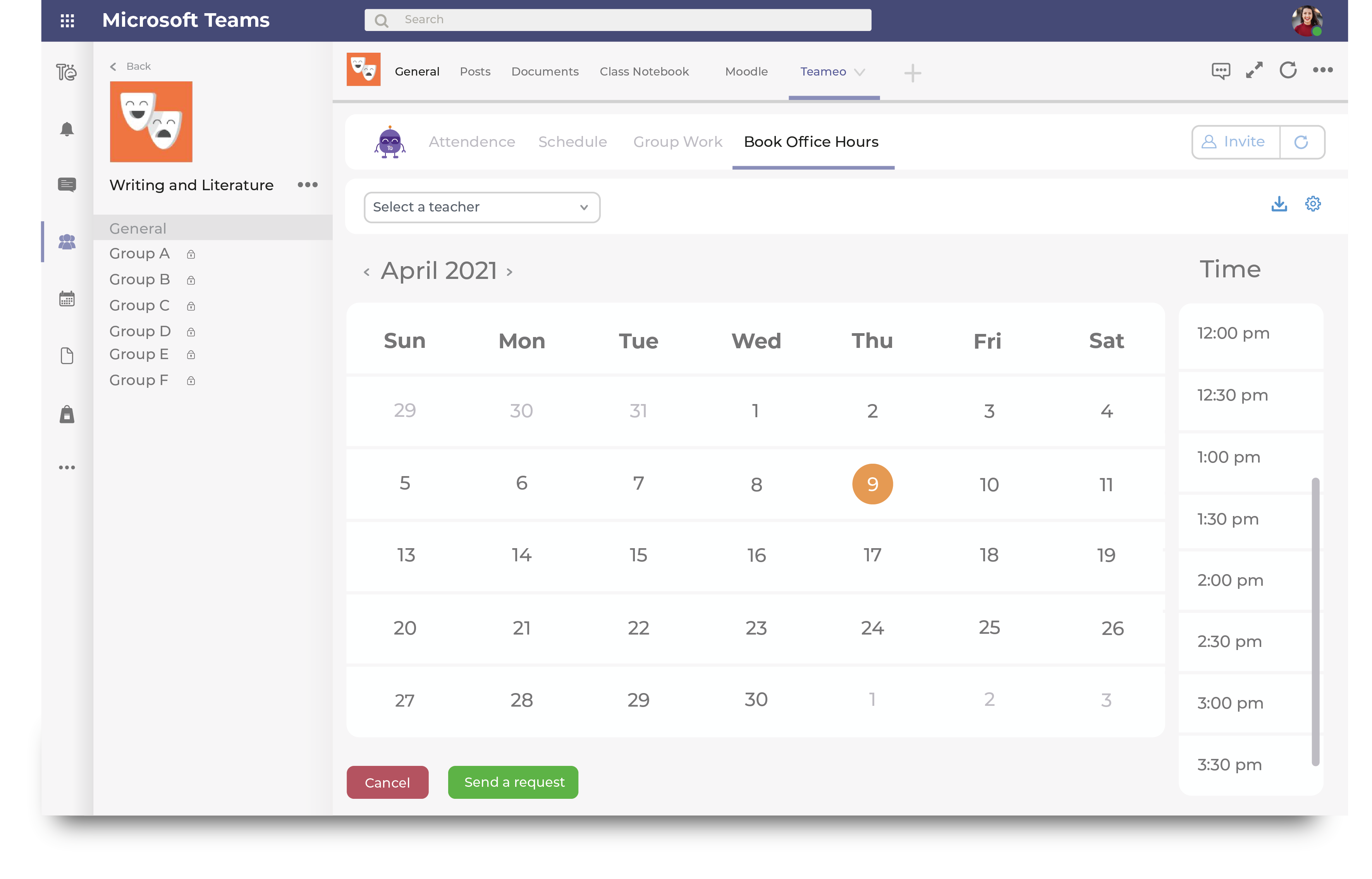Screenshot of a Microsoft Teams Scheduling Page

This screenshot captures a Microsoft Teams scheduling interface. The top of the page features a blue banner with the words "Microsoft Teams" in white font on the upper left corner. Centrally located on this banner is a search bar, and at the upper right corner, there is a small, indistinct profile picture.

On the left side of the interface, just below the banner, there's a square icon displaying a laughing and smiling mask figure, labeled "Writing and Literature." Below this, a vertical list categorizes various groups including General, Group A, Group B, Group C, Group D, Group E, and Group F.

Dominating the right side of the screen is a calendar for April 2021, with April 9th highlighted in vibrant orange. Positioned immediately above the calendar is a comprehensive menu offering several options: Attendance, Schedule, Group Work, and Book Office Hours.